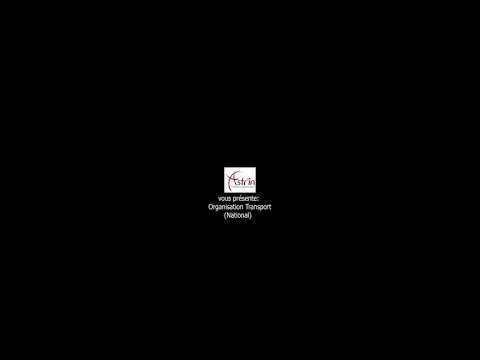The image features a completely black background with no gradations or lighter areas. At the center of this black square is a very small white square, comprising only about 5-10% of the total area. Inside this white square, there's a logo with the word "Astrin" written in small, pixelated red text. Below the logo, there's even smaller, almost illegible text. Directly beneath the white square, in slightly larger but still very small white letters, it says "Vouz Presentante, Organization Transport National," which is in French. This central area, resembling a desktop icon, is the focal point of the otherwise solid black image.